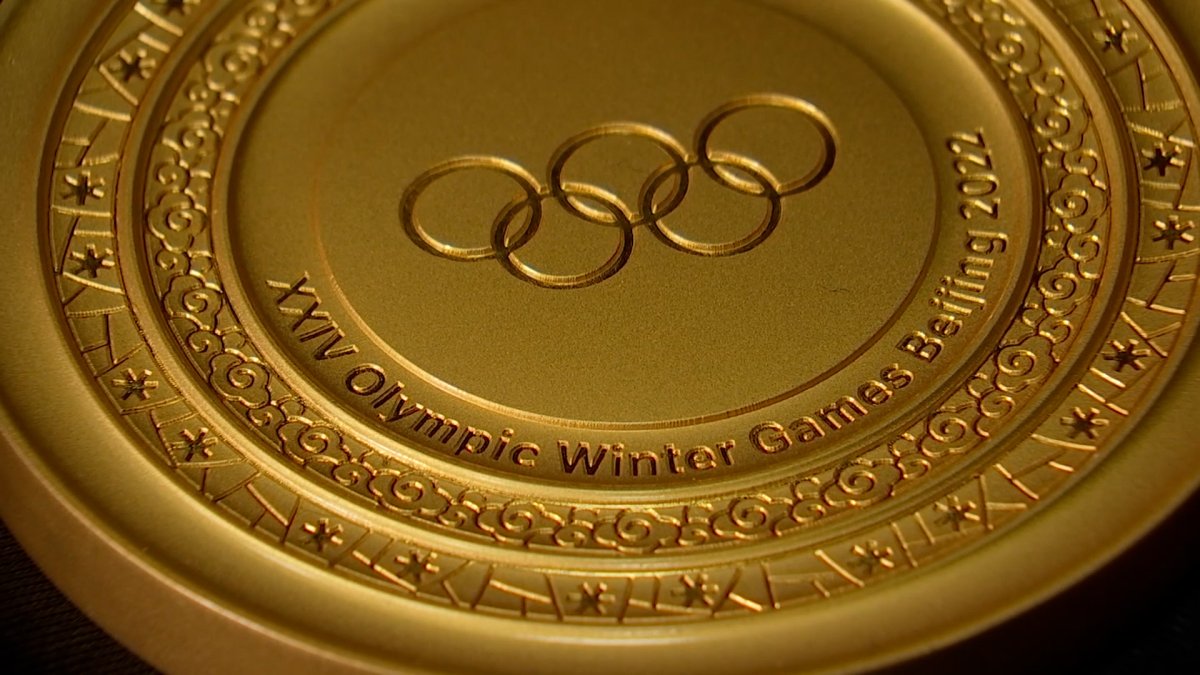The photograph is a close-up image of a gold Olympic medal from the 24th Olympic Winter Games held in Beijing in 2022. The medal is partially cropped and extends beyond the edges of the frame, set against a plain black background that likely represents a tabletop. The central focus of the medal features the five Olympic rings, stamped in monochrome. Surrounding this central emblem is an inscription in Roman numerals, spelling out "XXIV Olympic Winter Games Beijing 2022." The next ring is bordered with a design that some interpret as clouds and others as intricately embroidered flowers, possibly cherry blossoms. Beyond this decorative element is another ornamental ring composed of geometric shapes including stars and various intersecting lines. Additional raised rings on the medal contribute to its layered aesthetic, finishing with an unembellished outer edge. The entire medal, although possessing an illustrious gold hue, appears somewhat matte due to the lighting, which gives it a slightly plastic appearance in the photograph.